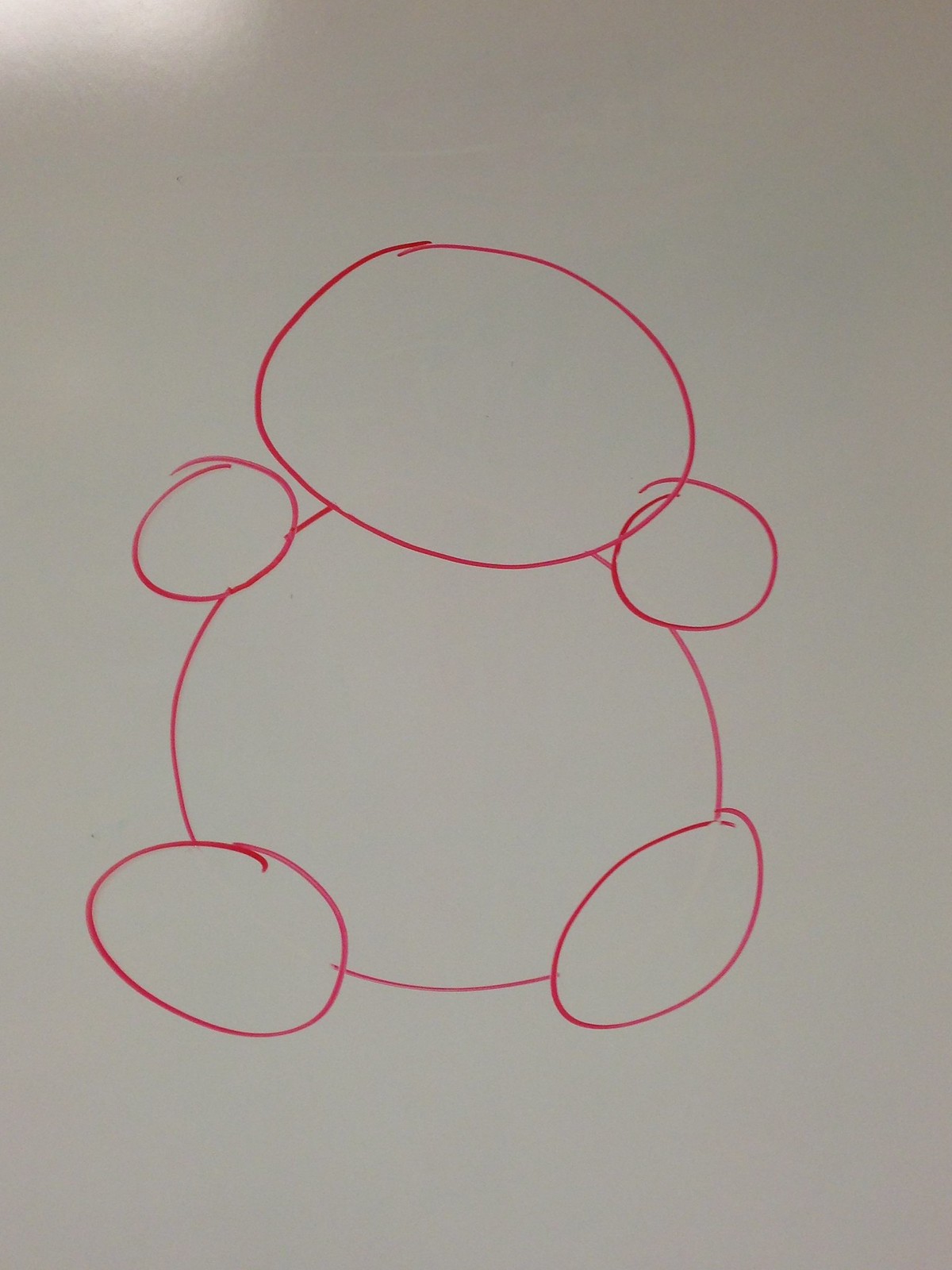A simplistic yet vivid marker drawing of a character is depicted on a white marker board. The character comprises distinct red circles: one at the top representing the head, two on either side for the hands, one in the center as the body, and two at the base for the feet. The surface of the board itself is a clean white with a gentle gradient towards a white-gray background. The upper left corner appears notably illuminated, adding an additional dimension of lightness to the scene. In the middle of this background rests the marker-drawn figure, standing out prominently with its bright red circular features. The overall composition is minimalistic, focusing on the fundamental shapes to bring the character to life.